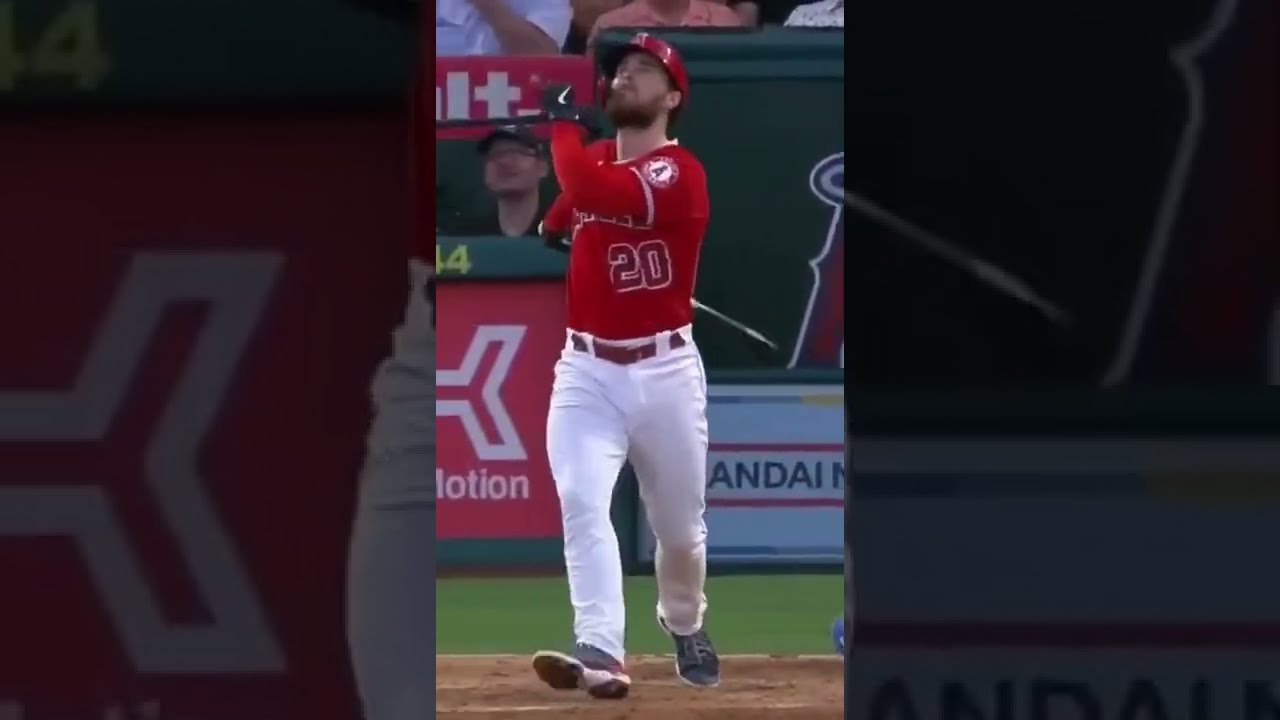The photograph captures a moment from a professional Major League Baseball game, specifically featuring a player from the Los Angeles Angels. The player, a white male with a thick ginger beard, is dressed in the team's uniform, which includes white tight pants, a red belt, and a red shirt adorned with a small 'A' on the sleeve and the number 20 in red lettering with a white outline. He sports a red baseball helmet and black gloves with a distinctive white Nike swoosh.

The scene appears to depict the player right after hitting the ball, as he is positioned at home plate with his right arm raised, hand gripping a black bat behind him, while his left arm lags slightly behind. His gaze is directed upwards and towards the top left corner, suggesting he is following the trajectory of the ball, possibly anticipating a home run. In the background, fans are visible, with one spectator in a baseball cap and glasses also looking in the same direction as the player. The dirt and elements of the stadium ground add to the dynamic atmosphere of the moment, marking it as an action shot filled with anticipation and energy.